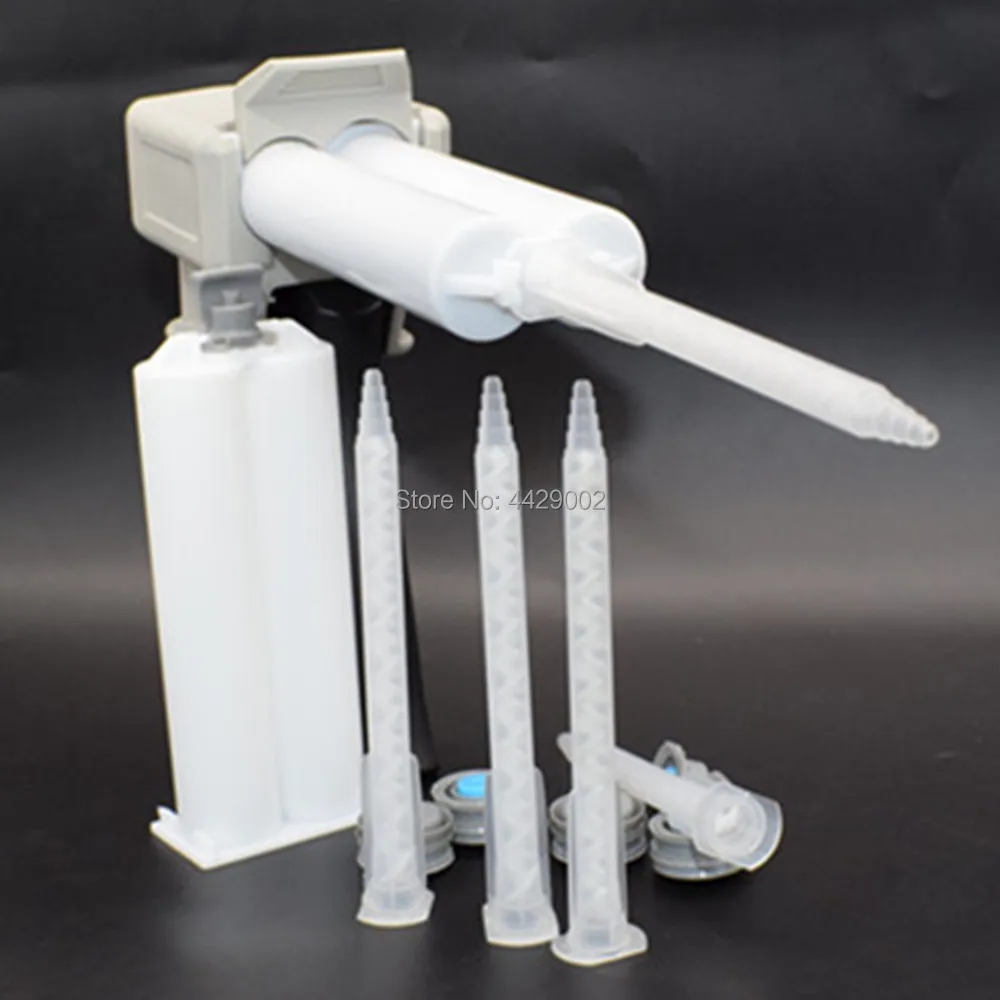The image depicts a medical or scientific device against a dark grey background, prominently featuring a watermark that reads "store number 4429002" at the center. The device consists of a white handle or base with a grey, cube-like rectangular prism attachment on top. Extending perpendicularly from this prism are two white cylinders that form part of the apparatus. Attached to the device is a translucent, pencil-shaped element resembling a tube of hot glue. Positioned vertically on the desk or surface below the main device are three additional translucent cylindrical objects. These cylinders, possibly made of plastic, stand upright with conical tips and oval-shaped flat bases. They each contain an intricate, zigzag straw-like pattern inside. The entire setup, predominantly in shades of white and pale grey, highlights the sleek design and functionality of the scientific tool.